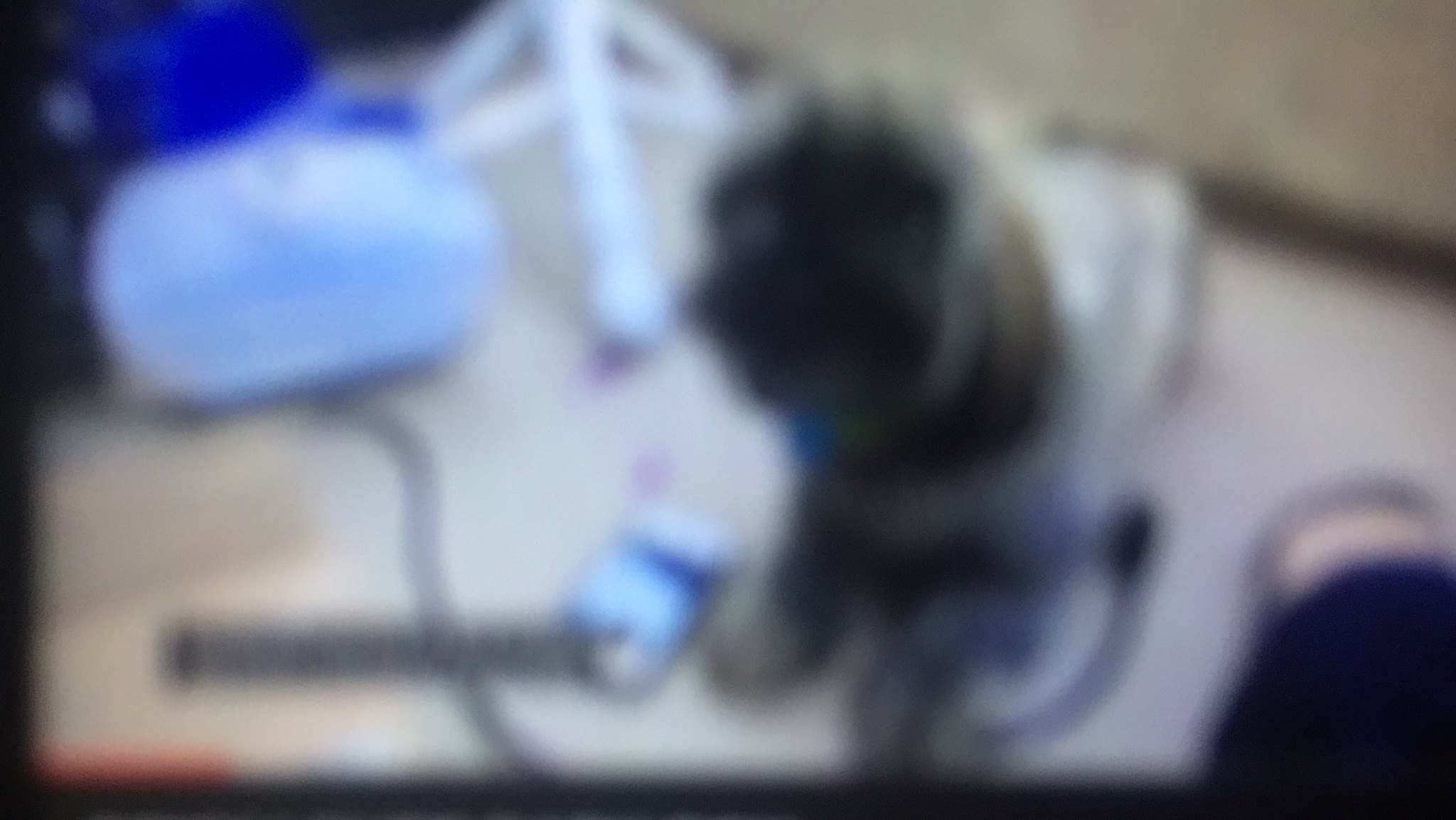The image appears to be a very blurred screenshot from a video, showing a gray-colored figure—potentially a dog or a statue of a dog—sitting on a white table. The figure, which has a blurry black face and short front legs, is positioned toward the left side of the frame, looking to the left from the viewer's perspective. The scene includes several objects: a white cylindrical container and long black wires underneath the table, along with a device featuring a blue screen, possibly a cell phone, and a long white piece with two white rectangles. The background is blue, and there is a white jog of some sort in the top left corner. Overall, the image's extreme blurriness makes finer details hard to discern, but it has an intriguing composition with scattered objects and the central figure.